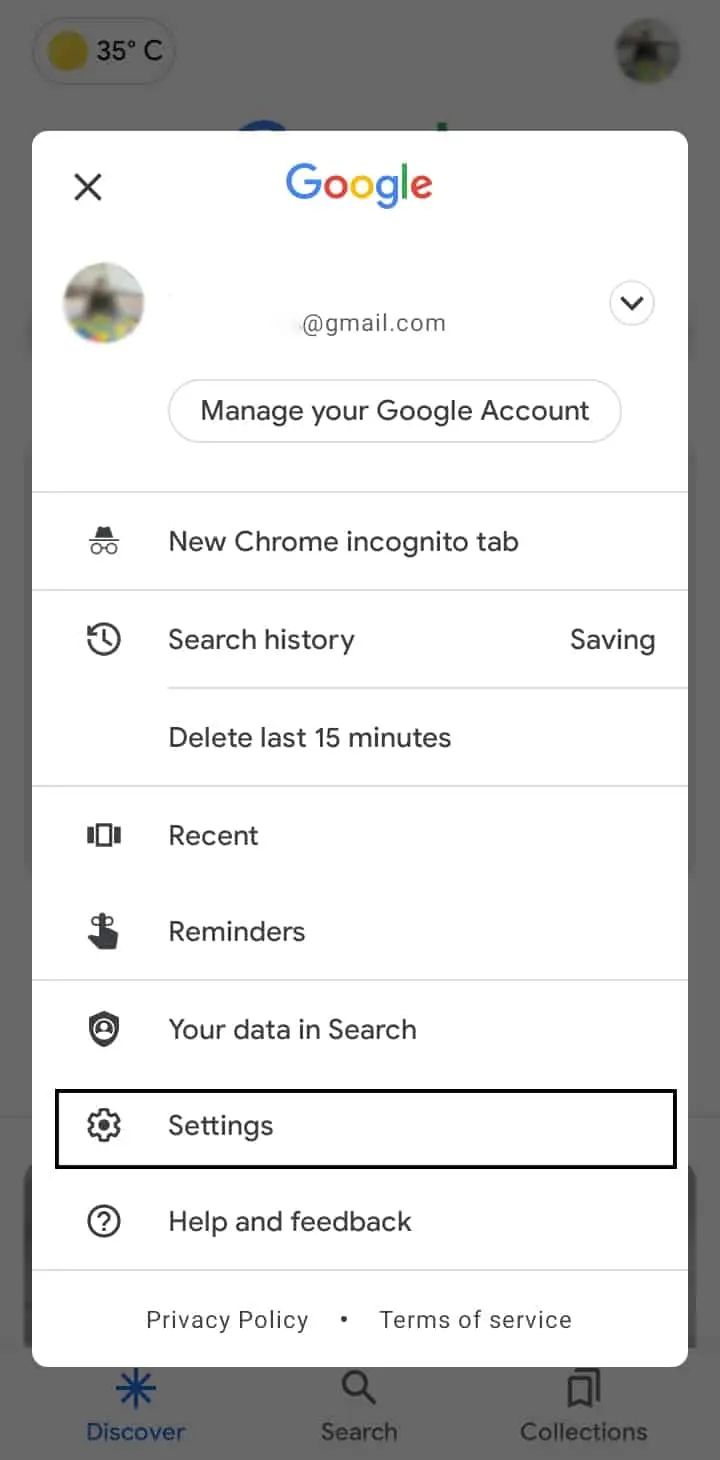The image displays a Google management panel on a smartphone, appearing as a pop-up screen overlaid with a white panel with curved corners. In the background, other elements on the phone are visible but mostly grayed out. The top left of the screen shows the current temperature as 35 degrees Celsius, while the top right features a blurred-out profile photo. Beneath these, the Discover, Search, and Collections options appear faintly at the very bottom.

The focal point is the white Google management panel. The panel includes a close "X" button in the upper left corner and the Google logo centered at the top. The same blurred-out profile icon reappears here, masking the user's Gmail address, showing only "blank white" and "@gmail.com," with a dropdown menu next to it.

Below the Gmail address, there is a "Manage your Google Account" option, followed by options to open a new Chrome incognito tab, indicated by an icon of a person wearing a hat and glasses. Next to it, a clock icon with a counterclockwise arrow signifies "Search history," along with options to "Save," and "Delete the last 15 minutes."

Further down are options for "Recent" and "Reminders," represented by various screen panels and an index finger tied with a bow. A shield icon symbolizes "Your data in Search." A highlighted gear icon indicates settings, marked with a black rectangle in this screenshot. A question mark inside a circle offers help and feedback, and at the very bottom, there are links to the "Privacy Policy" and "Terms of Service." Each option is separated by thin, one-pixel light gray lines.